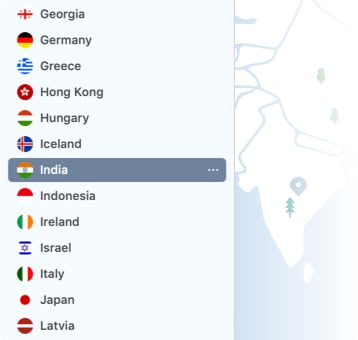This image is a computer-generated map in landscape format, rendered in full color. The map presents a very loose interpretation of global geography, with the oceans depicted in a light blue hue and the landmasses in white. The boundaries between regions are marked with soft, imprecise lines in shades of light blue and gray.

India is the most prominently featured country on the map, accompanied by its neighboring nations—Nepal, China, and Pakistan. Overlaying the map are small, rudimentary illustrations: a simple green and brown coniferous tree is located in central India, and pushpin symbols are scattered over China.

On the left side of the image, there's an alphabetical list of countries: Georgia, Germany, Greece, Hong Kong, Hungary, Iceland, India, Indonesia, Ireland, Israel, Italy, Japan, and Latvia. Within this list, 'India' is highlighted, indicating it's the country currently selected.